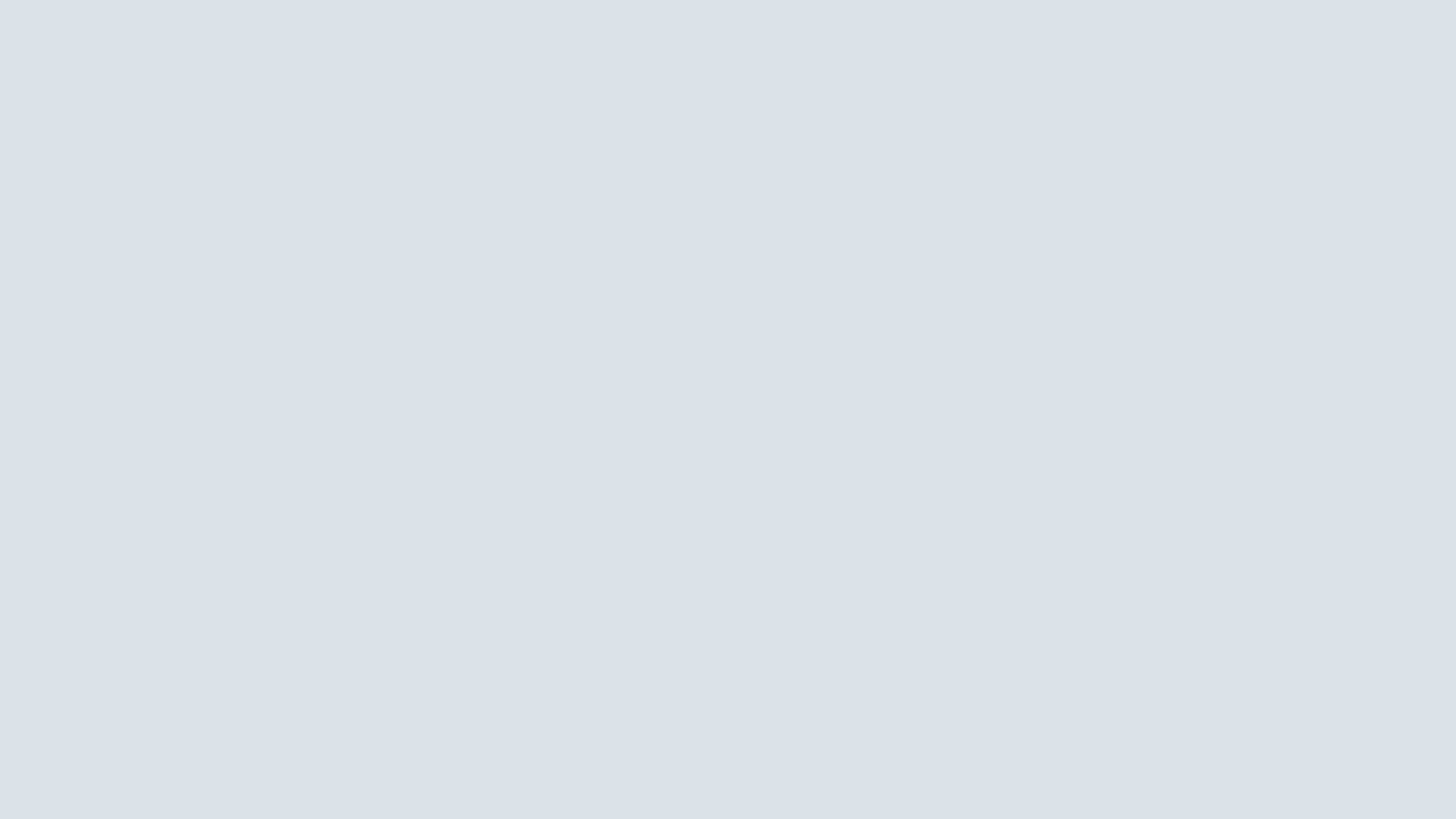This image showcases a pristine, long rectangular box against a backdrop of a light blue sheet. The box itself, a very light blue in color, is flawlessly even with precise squared corners. It bears no distinctive markings, print, or special features, presenting an immaculate and uniform appearance. Both the box and the background share a tranquil, pale blue hue, emphasizing the minimalistic and clean design of the composition.